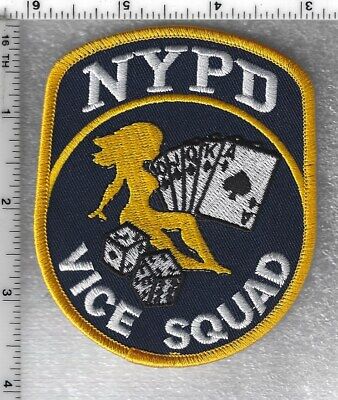This image depicts a humorous embroidered patch designed to mimic a New York Police Department (NYPD) Vice Squad badge. The patch is bordered by a golden-yellow trim and features a dark navy blue background with intricate details. At the top, in a semi-circular arrangement, the letters "NYPD" are embroidered in white. The central circular section showcases several elements: a seductive golden-yellow outline of a woman, a white and black rendition of a royal flush in spades, and a pair of dice displaying a 3 and a 4. Below these visuals, the words "VICE SQUAD" are prominently embroidered in capital letters. The patch is displayed against an off-white background, accompanied by rulers indicating its size, approximately three inches wide by four inches tall. The top ruler measures up to 6 1/4 inches (upside down), while the left ruler extends to just over 4 inches, with each line representing 1/16 of an inch.